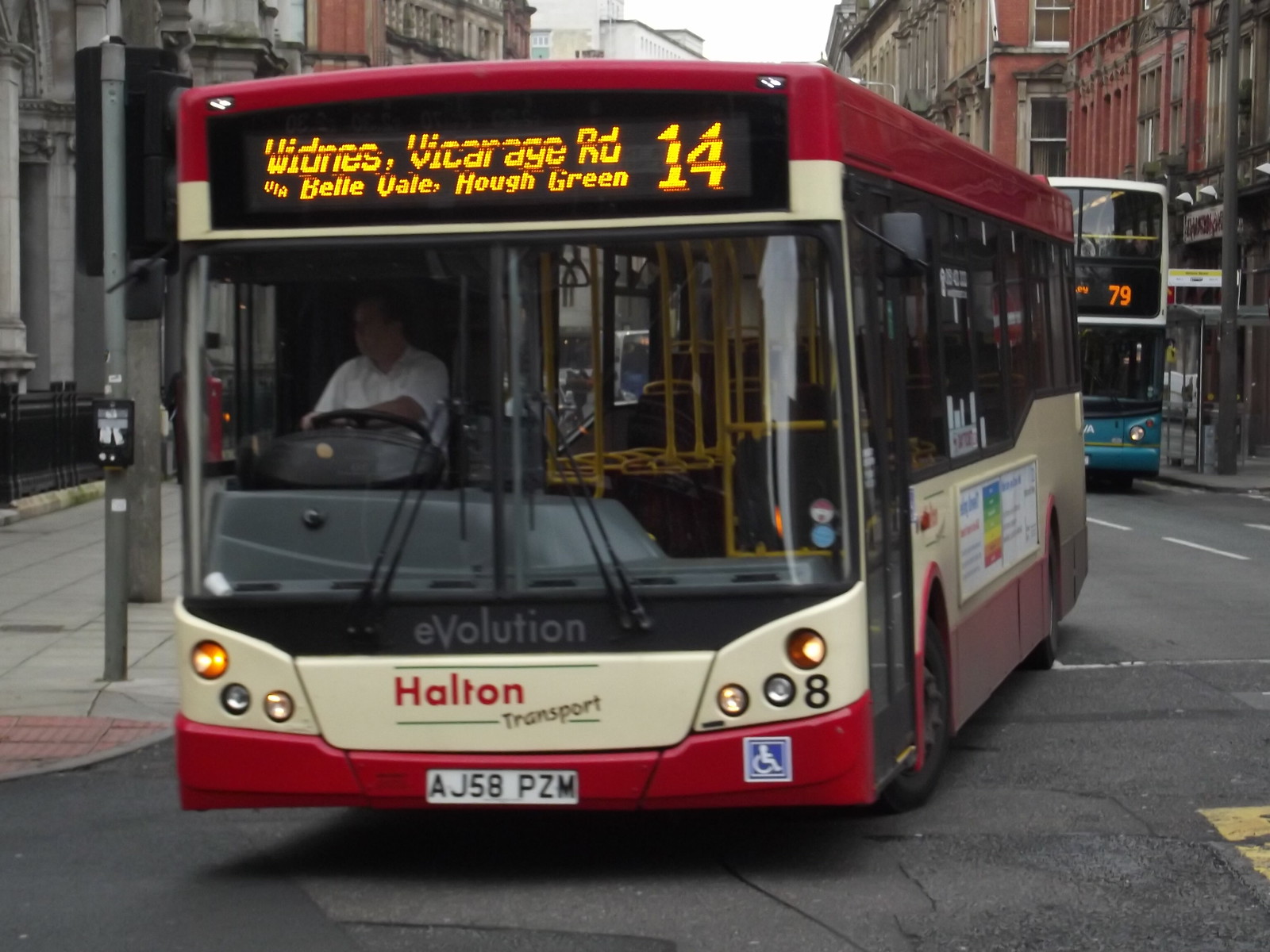The image captures a public transportation bus, predominantly red with a white band wrapped around it, driving towards the camera on a city street lined with buildings on the left and right, and parking meters to the left. The bus is identified as a Halton Transport vehicle, its front bumper featuring a red hue with a license plate reading AJ58PZM and a handicap sign positioned on the right side. Prominently displayed above the bumper are the words "Halton Transport" in white lettering, flanked by headlights. The bus is designated as number 14, with an upper electronic ticker indicating its route: "Widness, Vicarage Road, Belle Vale, Ho Green." This sign features yellow text on a black background. The top border of the bus is red and the bus bears the term "Evolution" in white letters on a black background above the main signage. Inside, yellow railings are visible, but the bus appears empty, with the driver, dressed in a white shirt, seated on the left. Another double-decker bus, predominantly blue on the bottom, can be seen behind it, suggesting a busy urban environment. The buses seem to be navigating a turn, with the red and white bus turning right, situated on the left-hand side of the image.